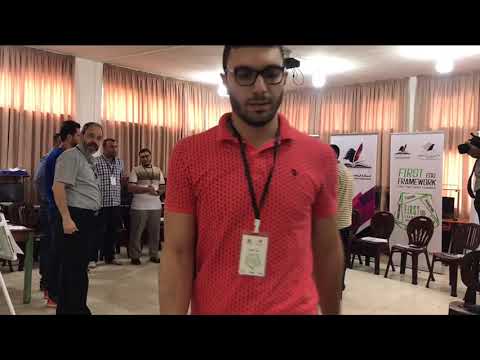This image captures a close-up of a man standing at the center, facing the camera, clad in a reddish-pink polo shirt with a lanyard around his neck. The lanyard has black strings and appears white, but the text on it is unreadable due to the blurriness. The man, who has dark hair, a dark beard, and mustache, and is wearing dark-framed glasses, is visible from his head down to his waist. He seems to be looking slightly downward. The setting seems to be a conference or some learning event, as evidenced by the other men in the background, also wearing lanyards and either standing or talking among themselves. Chairs are arranged in a circular or scattered manner, and on the right side of the image, several signs are visible, including one that states "First Framework," although it's somewhat blurry. The room is surrounded by curtains concealing windows that allow sunlight to filter in, giving clues to an attempt to keep the room cooler and darker for the meeting. There are also noticeable ceiling lights adding to the indoor illumination. On the far right, the edge of another person holding a camera is faintly visible.